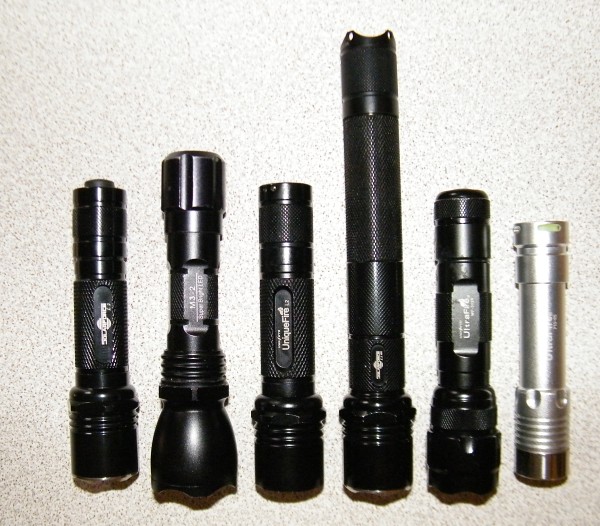This image depicts six tactical flashlights of various sizes arranged on a speckled white and gray surface. Five of the flashlights are black, and one is silver. They are mostly crafted from heavy-duty metal, which feels cold to the touch. Two of the flashlights prominently display the brand name "Unique Fire," while another has partially readable text that appears to say "ultra flex." The flashlights vary in length; the fourth one from the left is the longest, standing about five inches taller than most others, while the silver one is the shortest. The flashlights seem to be laying down, given the shadow cast beneath them at the point where the light exits. This assortment includes gear suitable for tactical use, with some potentially serving as everyday carry options.